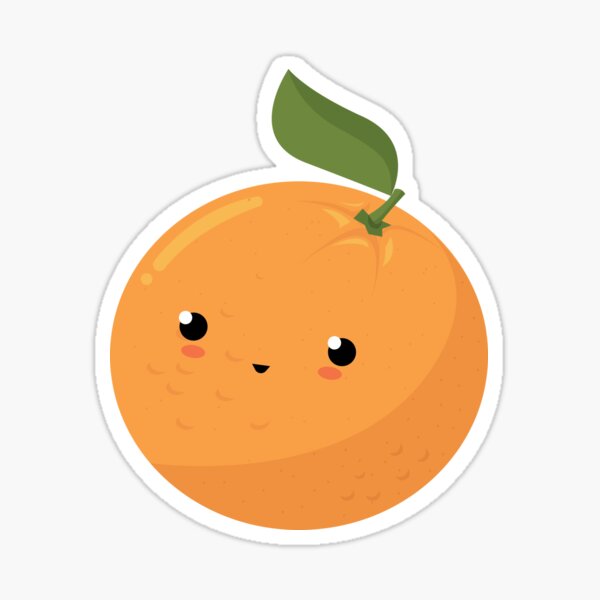This image depicts a cute, cartoonish sticker of an orange, possibly resembling a small tangerine like a Cutie. The orange has a round shape with a single green stem protruding from the top at a slight angle, accompanied by a two-toned, darker and lighter green leaf. The orange features a smiling face with two dark eyes highlighted by white dots for a lifelike appearance, tiny rosy cheeks, and a small, smiling mouth directly beneath the eyes. The orange's surface includes lines indicating dimples and shading—darker at the bottom half—suggesting the effect of light and shadow. The entire image is outlined in white, reinforcing the sticker-like quality, and the background of the scene is also white.